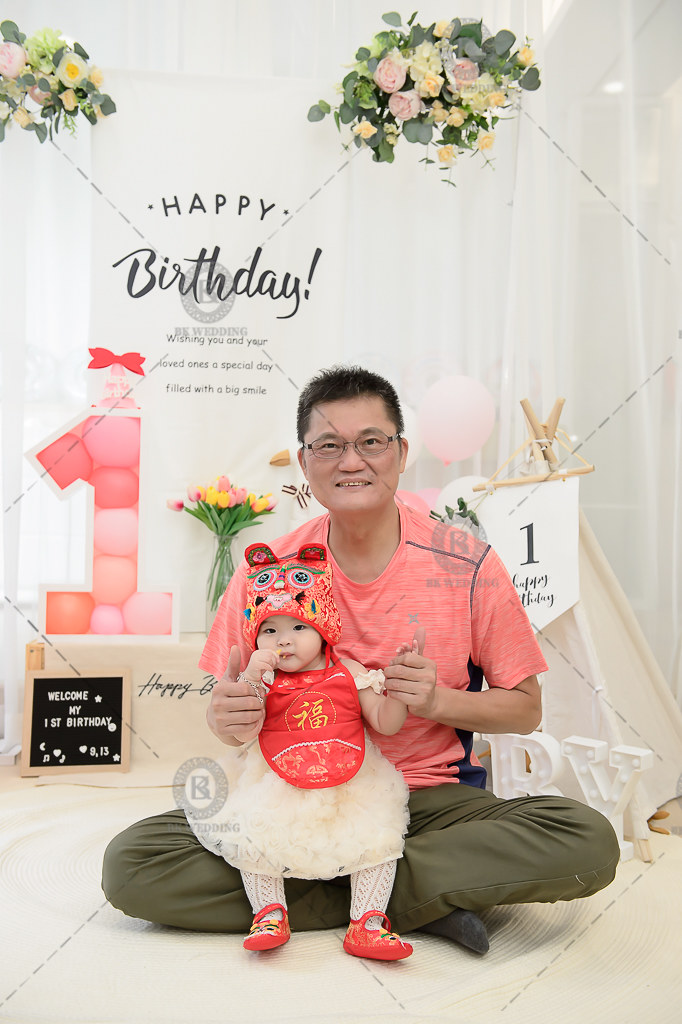The image captures a festive first birthday celebration featuring a father and his daughter, both of Oriental descent. The father, who has glasses and short dark hair, is dressed in a peach-colored short-sleeve shirt and tan pants, and is sitting cross-legged while holding his daughter on his lap. The little girl is adorned in a white dress with a red bib, a hat with red ears, and red shoes. Surrounding them is a colorful backdrop comprising yellow and pink floral arrangements. A prominent banner behind them reads "Happy Birthday" with a lengthy vertical sign featuring a large pink number "1." Below this, a chalkboard conveys the heartfelt message "Welcome My First Birthday." The entire scene is rich with celebratory details, making it a perfect depiction of a joyful birthday greeting card or poster for the baby's milestone.